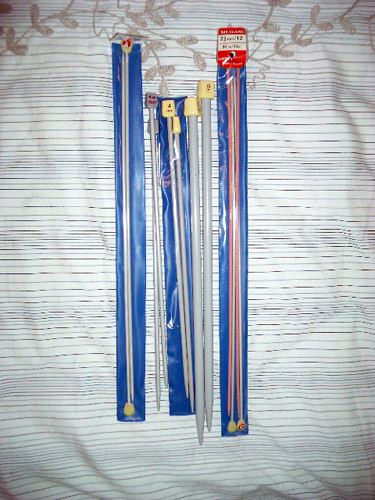This image is a detailed photograph of various knitting needles laid out on a grey fabric backdrop, adorned with subtle horizontal brown lines and embroidered leaf designs. The knitting needles are arranged in pairs, with some housed in transparent blue containers. Among the needles in the containers, one on the right features a red and white tag with indecipherable black text, enclosing both grey and red needles. Centered in the image, two needles have distinctive yellow tips and are placed in another blue case. The needles vary in color and material; some are opaque, clear, red, or grey. The fabric beneath the array of needles provides an elegant contrast with its finely striped texture, punctuated by thicker stripes and embroidered brown leaves, adding a touch of design flair to the setting.